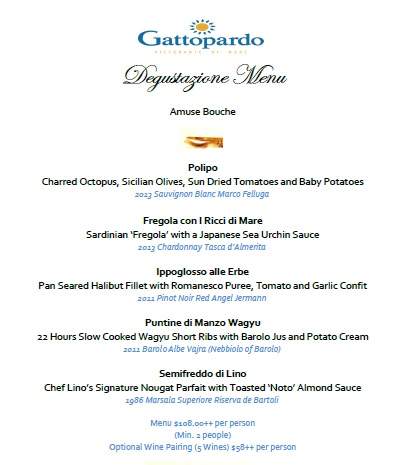The image showcases a sophisticated menu from the restaurant Gatto Pardo, against a white background. At the top, the restaurant’s name, "Gatto Pardo," is prominently displayed in blue font. Below it, in elegant gold writing, is the title "Degustazione Menu." The menu begins with an "Amuse-Bouche," and proceeds with several detailed courses:

The first course is "Polipo," featuring charred octopus, Sicilian olives, sun-dried tomatoes, and baby potatoes, paired with a 2013 Sauvignon Blanc from Marco Falugo. The second course, labeled "Frigula conrici de mer," includes Sardinian frigola with a Japanese sea urchin sauce, accompanied by a 2013 Chardonnay from Tasca d’Almerita. 

Next is "Hipoglosso alla piastra," a pan-seared halibut fillet with Romanesco puree, tomato, and garlic confit, paired with a 2011 Pinot Noir, ‘Red Angel’ from Jermann. Following this, "Pancia di manzo" consists of 22-hour slow-cooked Wagyu short ribs with Barolo jus and potato cream, accompanied by a 2011 Barolo from Alba Vajra Nebbiolo.

For dessert, the "Semifreddo di Lino" presents Chef Lino’s signature nougat parfait, topped with toasted Noto almond sauce, paired with a 1986 Marsala Superiore Riserva from De Bartoli.

The menu is priced at $108 per person, with a minimum of two people required. Optional wine pairing is available, featuring five wines, for an additional $58 per person.